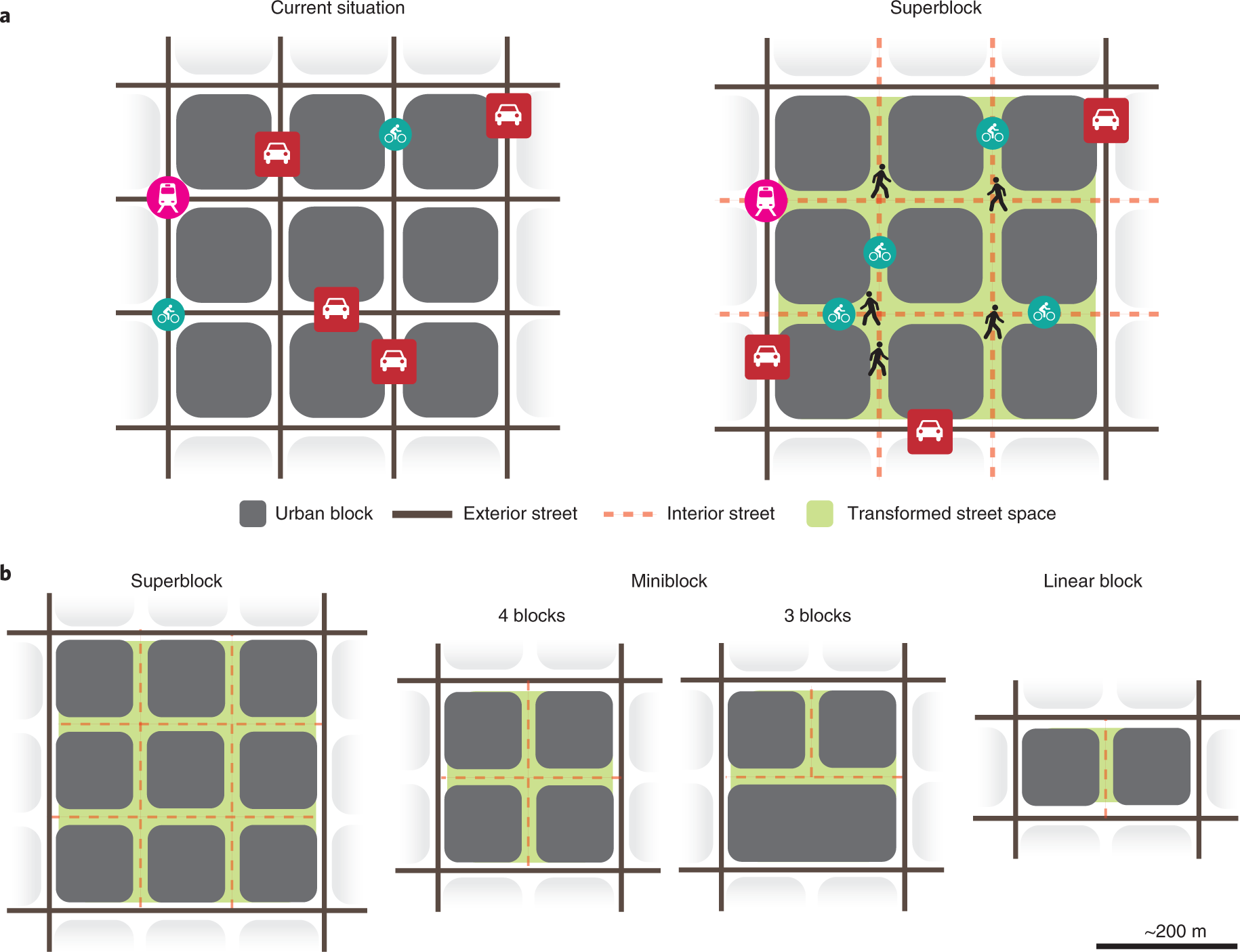The image is a detailed diagram illustrating urban block layouts, traffic patterns, and the concept of a "Superblock." At the top, two grids each labeled with "Current Situation" and "Superblock" respectively, depict nine gray squares representing urban blocks. 

In the "Current Situation" grid, four mini red squares marked with white car symbols are located in different sections of the grid, indicating car presence. A pink vehicle is shown on the far left, surrounded by small bluish teal symbols, depicting various transportation icons. The grid has gray rounded squares within each sub-square, delineating the interior space.

The "Superblock" grid features nine similar gray rounded squares, but with lime green areas representing transformed street spaces, where the thin gray lines signify exterior streets and red dotted lines mark interior streets. This grid also has symbols of people walking and teal transportation icons, indicating a shift towards pedestrian and non-motorized traffic in the central parts, confining cars to the periphery.

Below these primary grids are four progressively smaller grids labeled "Superblock," "Four Blocks," "Three Blocks," and "Linear Block." Each grid decreases in complexity, with the smallest depicting a single linear arrangement of blocks. This visualization underscores the transition from smaller, individual blocks to a conceptually larger, integrated superblock system, reducing car traffic and enhancing pedestrian spaces.